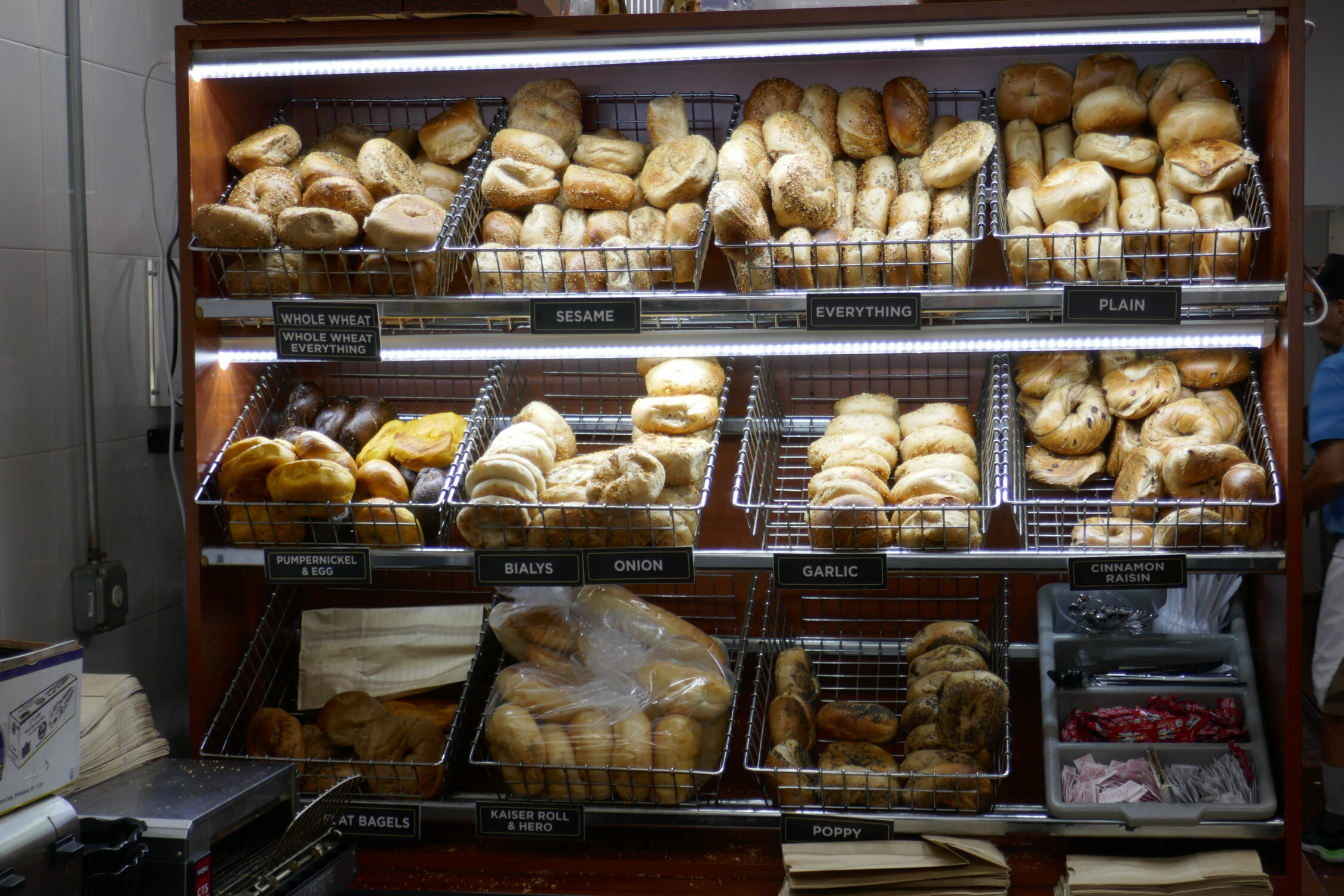The photograph captures the interior of a bagel shop, showcasing an organized display of various bagels in wire baskets arranged on three shelves. Each shelf features a different assortment, with the top two shelves each holding four baskets, while the bottom shelf has three. The bagels are distinctly labeled with flavors including whole wheat, whole wheat everything, sesame, everything, plain, pumpernickel, egg, Bailey's, onion, garlic, cinnamon, raisin, wheat or oat bagels (partially obscured), kaiser rolls, and poppy seed. The wire baskets are angled at approximately 45 degrees for easy viewing. Surrounding this display, there are several condiments in a gray container, paper bags stacked near the shelves, and metal items such as a tin table for cutting bagels and possibly a toaster or scale. Additionally, plastic bags with bagels inside are seen on the bottom. Above all, the setup, combined with the long pole with an electrical outlet, suggests a busy and well-stocked bagel shop.